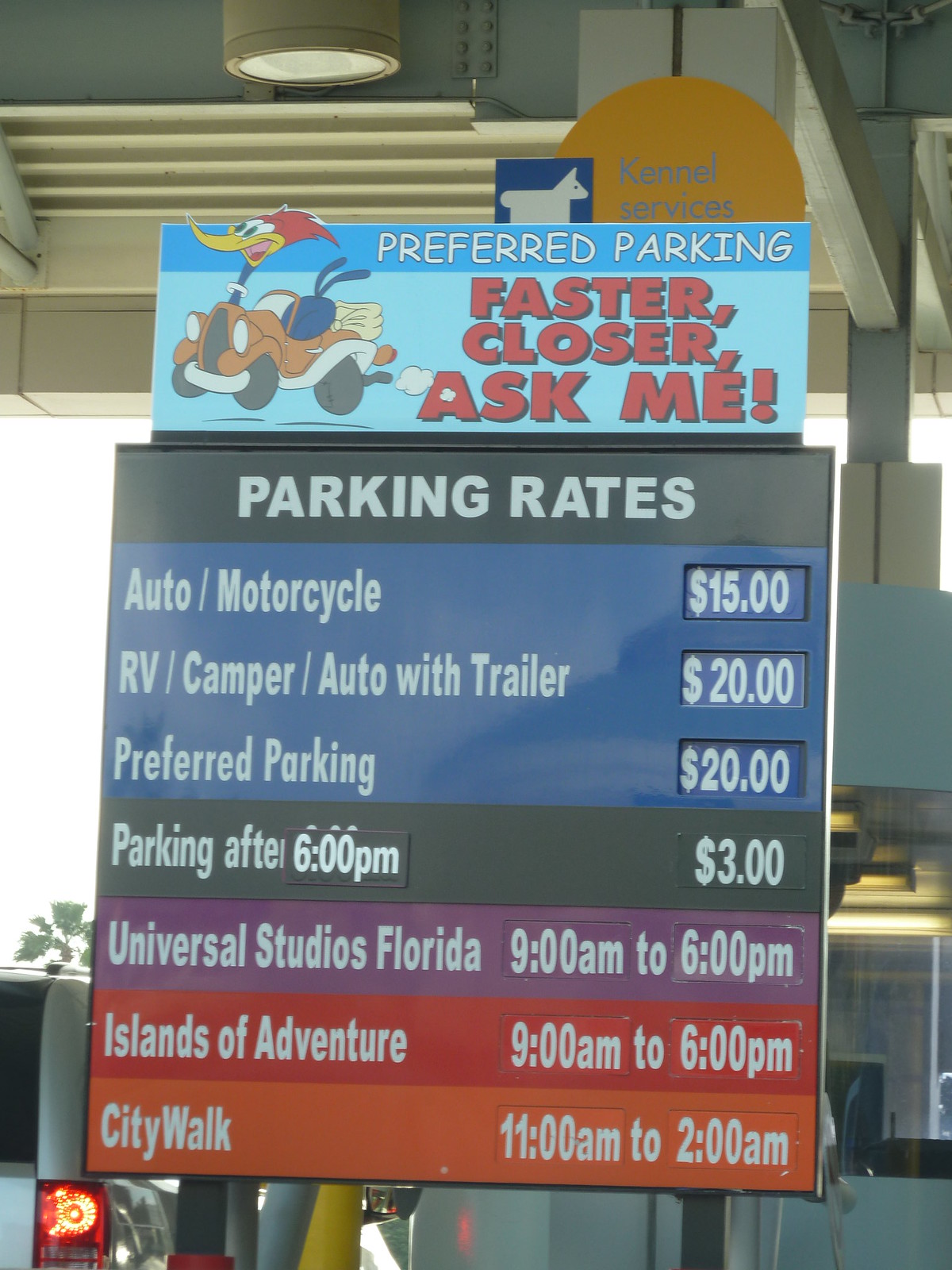The image captures a daytime scene with the top of a building visible in the background. Hanging from a covered area is a detailed informational sign that displays parking and operational details. At the top, the sign promotes "Preferred Parking: Faster, Closer, Ask Me" with an illustration of Woody Woodpecker in a car pointing to the left, and a section above indicating "Kennel Services" with a white dog icon. Below in a blue box with white font, the parking rates are listed: "Auto/Motorcycle - $15, RV/Camper/Auto with Trailer - $20, Preferred Parking - $20." Beneath this, in a black box, the rate for parking after 6 p.m. is stated as "$3." Further below, the operating hours for various attractions are displayed in colorful rectangular boxes: "Universal Studios Florida 9 a.m. - 6 p.m." in a purple box, "Islands of Adventure 9 a.m. - 6 p.m." in a red box, and "City Walk 11 a.m. - 2 a.m." in an orange box.